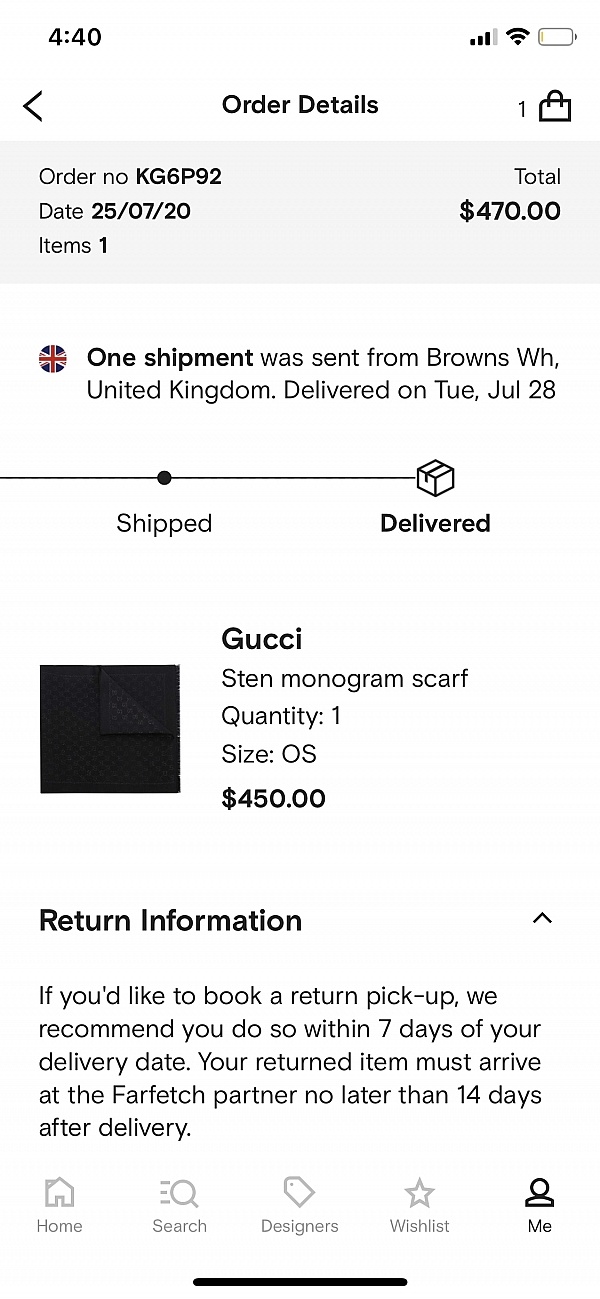The image depicts a smartphone screen displaying an order summary and delivery details. 

On the left, there is an icon indicating cellular signal with "4G" displayed. To its right, there are icons showing Wi-Fi connectivity and battery status, with the latter nearly depleted and colored slightly yellow. At the bottom of the screen, a left-facing arrow is positioned on the left, prominently in the center is "Order Details," and to the right is a shopping bag icon displaying the number "1."

Below this header, the order number "KG6P92" is shown. Following this, it shows "Date: 25/07/20" and "Items: 1," while on the right, the total amount is listed as "$470."

A British flag icon indicates the delivery destination: "One item shipped to Browns WH, United Kingdom," with delivery completed on "Tuesday, July 28th." A timeline below marks the shipping and delivery status, ending with a package icon labeled "Delivered."

The item summary lists a "Gucci Sten Monogrammed Scarf" with "Quantity: 1" and "Size: OS," priced at "$450." 

The return policy advises booking a return pickup within seven days of delivery, and ensuring the item reaches the Farfetch partner no later than 14 days post-delivery.

At the bottom of the screen, there is a navigation strip with icons labeled "Home," "Search," "Designers," "Wishlist," and the current selection highlighted as "Me," which is darkened while the others remain gray.